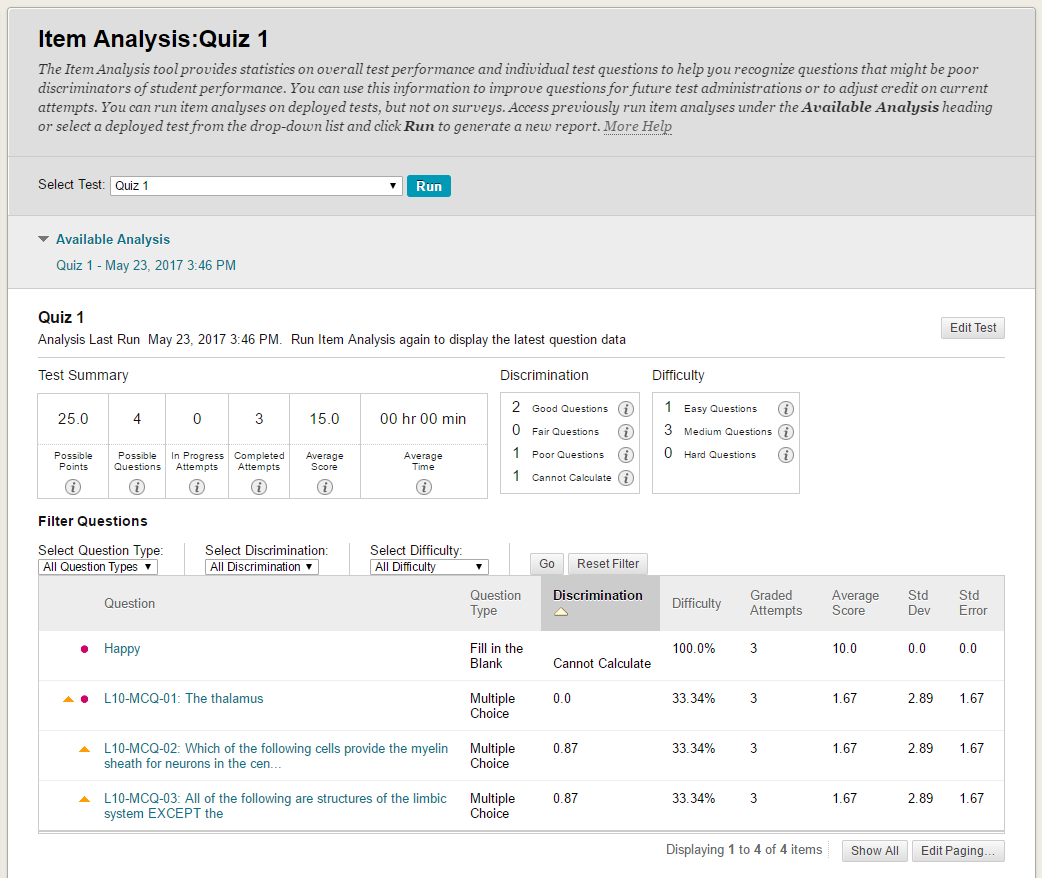This image depicts a detailed screenshot of a web-based analysis tool used for evaluating quiz performance. The primary layout comprises a tannish border that extends across the top and sides of the page, but not at the bottom, creating a partial frame. Inside this border, a thin gray line further delineates the boundaries, also excluding the bottom edge. 

At the top of the image, there is a dark gray box situated in the upper left corner, highlighted against the background. This box prominently displays the title "Item Analysis: Quiz One." Below this title, a description is provided, stating: "The item analysis tool provides statistics on overall test performance and individual test questions to help you recognize questions that might be poor discriminators of student performance." It also includes instructions on various functionalities such as selecting "Test Quiz One" and pressing "Run" to initiate the analysis.

Further down, a section in teal shows, "Available Analysis - Quiz One, May 23rd, 2017 at 3:46 p.m.," providing the date and time when the last analysis was performed. It suggests running the analysis again to update the latest question data.

The tool then presents a comprehensive summary of the test, which includes metrics like "Discrimination," and "Difficulty." Additional options for filtering questions are available. Detailed information is provided for each question, including attributes such as the question title, type (e.g., fill in the blank), discrimination index, difficulty level, number of graded attempts, average score, student development insights, and error rates.

The display section shows items ranging from one to four out of a total of four questions, with options to view all items at once or edit the paging settings.